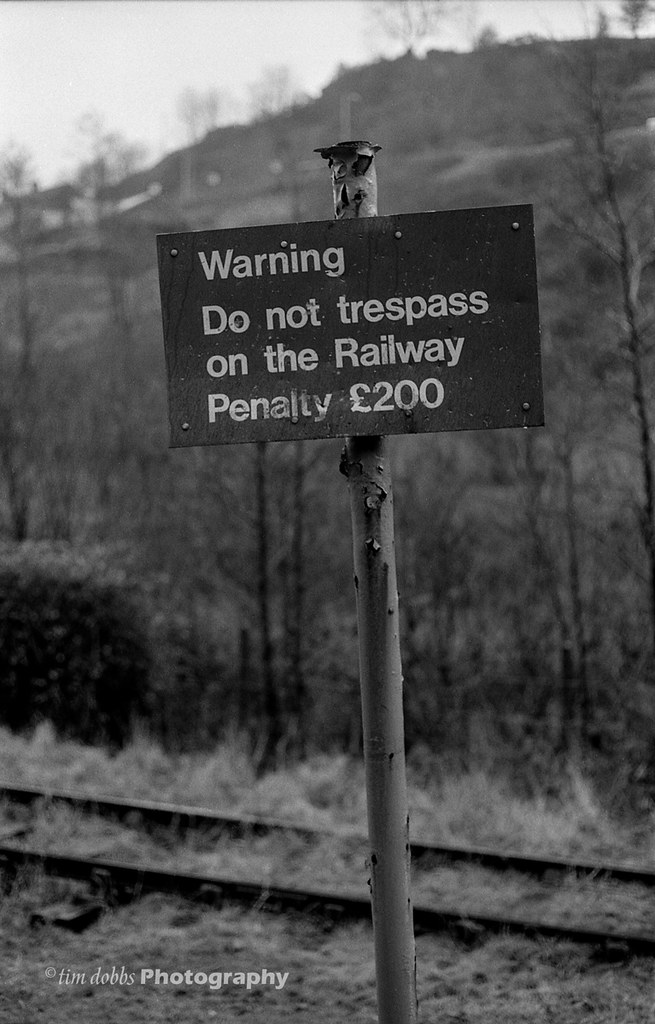This image is a black-and-white photograph titled "Tim Dobbs Photography," indicated by a watermark in the lower left corner. The scene captures an outdoor railway setting. Dominating the foreground is a dark sign affixed to a tall steel post, approximately five to six feet in height. In white, sentence-case letters, the sign reads, "Warning: Do Not Trespass on the Railway. Penalty 200 Pounds." The railway tracks run along the bottom of the image, partially obscured by overgrown weeds. In the background, there are leafless trees and a tall hill covered in grass and slim, barren trees, suggesting a fall or winter season. The overall composition is stark and plain, highlighting the desolation and simplicity of the rural landscape.